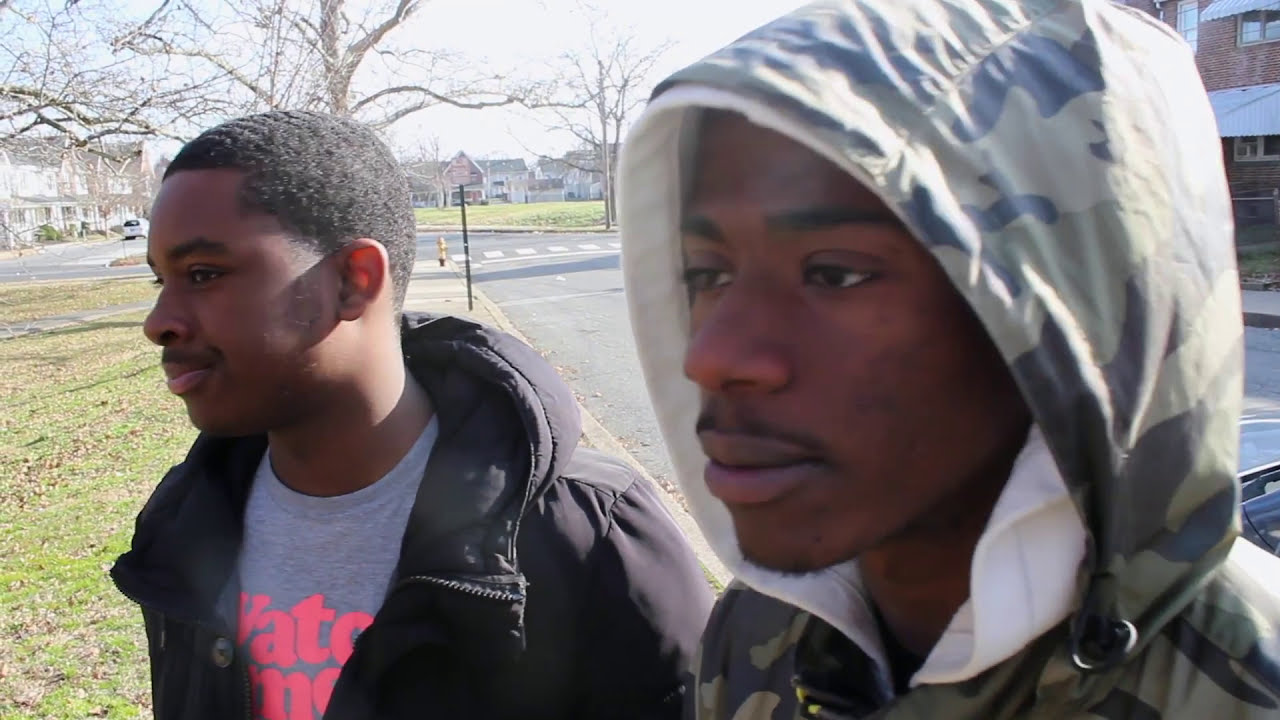In a sunlit, wintry residential area, two young black men stand on a grassy curb at the edge of a street. The street curves into the background, bordered by buildings on both sides, including tall, two-story wooden structures on the left and possibly a newer concrete building on the right. The bare branches of a tree frame the upper left of the image. The man on the right, facing left with sunlight illuminating his camo hood, wears a camouflage-patterned hoodie layered over another white-hooded shirt. The man on the left, also facing left, sports a black hooded jacket with the hood down, revealing a gray shirt adorned with bright pink lettering, partially displaying "WITC" and "ME." The background appears calm with minimal traffic, albeit a white car is parked near the street's edge on the far right.